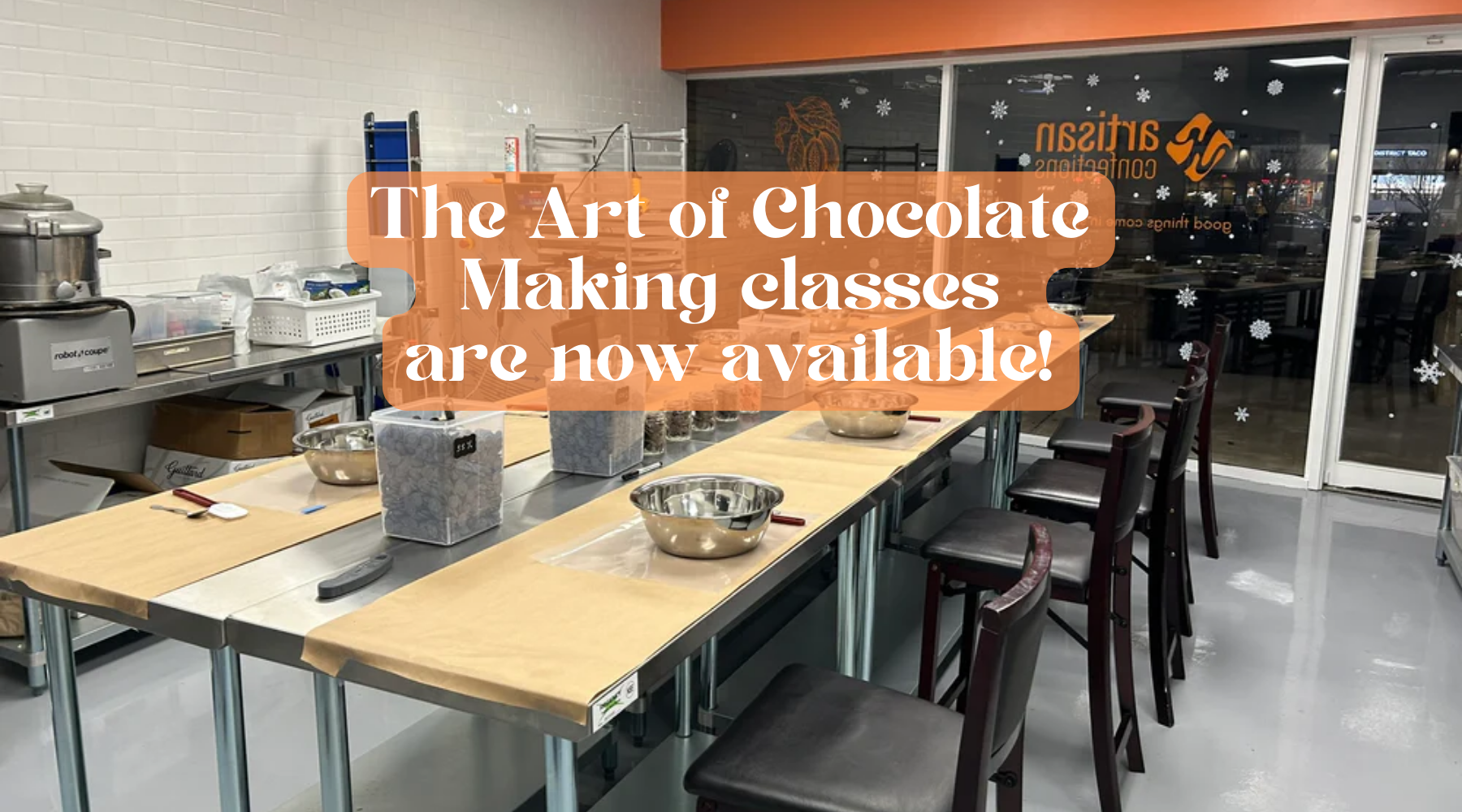The photograph features a detailed kitchen scene promoting "The Art of Chocolate Making Classes," as written in white text on a transparent orange overlay centrally placed in the image. The setting appears to be within an industrial kitchen or culinary classroom. A prominent, centrally located wooden table equipped with a stainless steel strip is prepared for chocolate-making activities, displaying various stainless steel mixing bowls, utensils, and jars presumed to contain chocolate pieces. Surrounding the table are four chairs with wooden frames and dark, cushioned seats.

To the left, a stainless steel counter holds an array of professional kitchen equipment, including a large mixer and multiple trays of utensils. Additional kitchen tools and cardboard boxes are organized on metal racks that hint at a busy yet structured environment. The far left side of the scene is marked by a white-painted brick wall.

In the backdrop, glass windows adorned with snowflake decals and transparent orange logos hint at festive preparations. The windows open into a storefront area, which, combined with the predominantly gray and shiny tile floor, adds a welcoming touch to the culinary workspace. The overall setup, underscored by the orange wall that connects the windows, radiates readiness and excitement for the chocolate-making classes to commence.